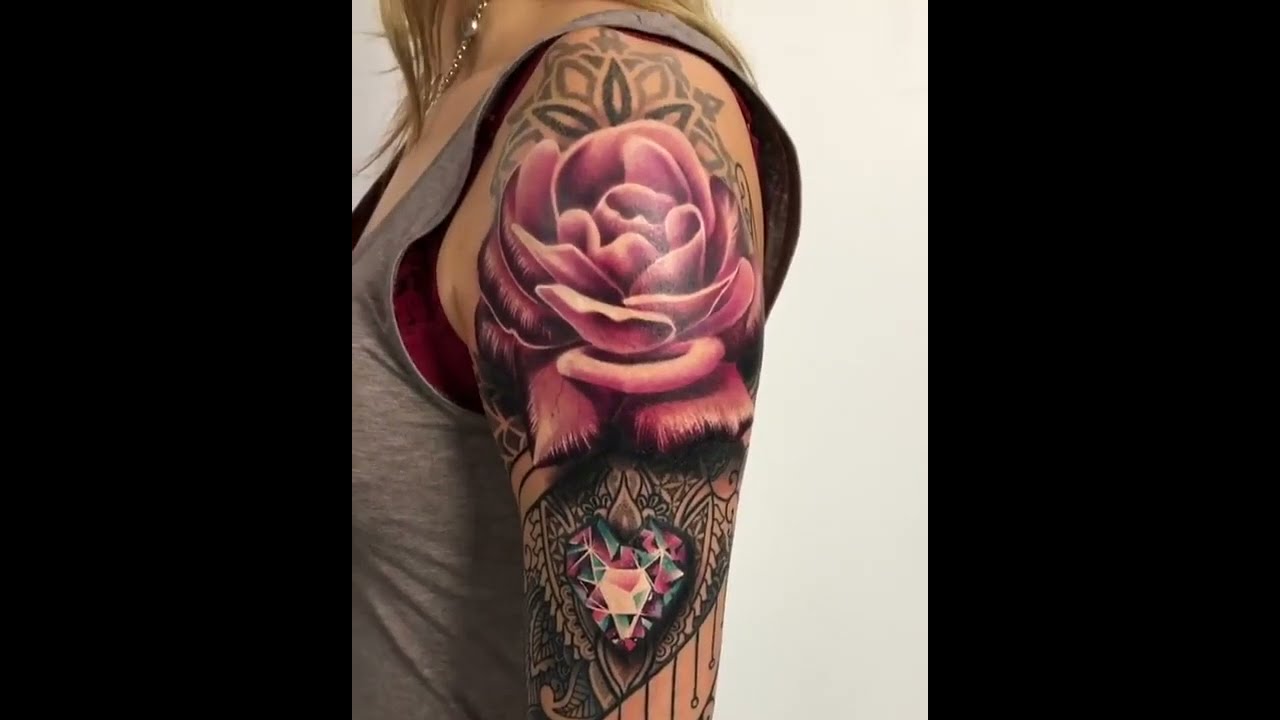The image features a three-panel design with the left and right panels completely black, framing the central rectangular photograph. Against a white background, a woman is shown in profile from her neck down, with her head cropped out of the frame. She has medium-length, slightly past-the-shoulders blonde hair and wears a silver chain necklace. Her clothing consists of a burgundy bra beneath a gray tank top, both sleeveless. The entire left arm is exposed, revealing a large, intricate tattoo. 

Her tattoo starts with a vivid pink rose on her shoulder, displaying dense petals with a backdrop featuring a dark green mosaic pattern. This mosaic design continues below the rose, incorporating dark gray and light gray outlines of leaves or petals. Below the rose, the tattoo transitions into a heart-shaped design that resembles a gemstone, with glistening, sharp-edged facets in teal and dark pink colors. A delicate, black lacy trim outlines the heart, adding to the complexity and elegance of the tattoo.